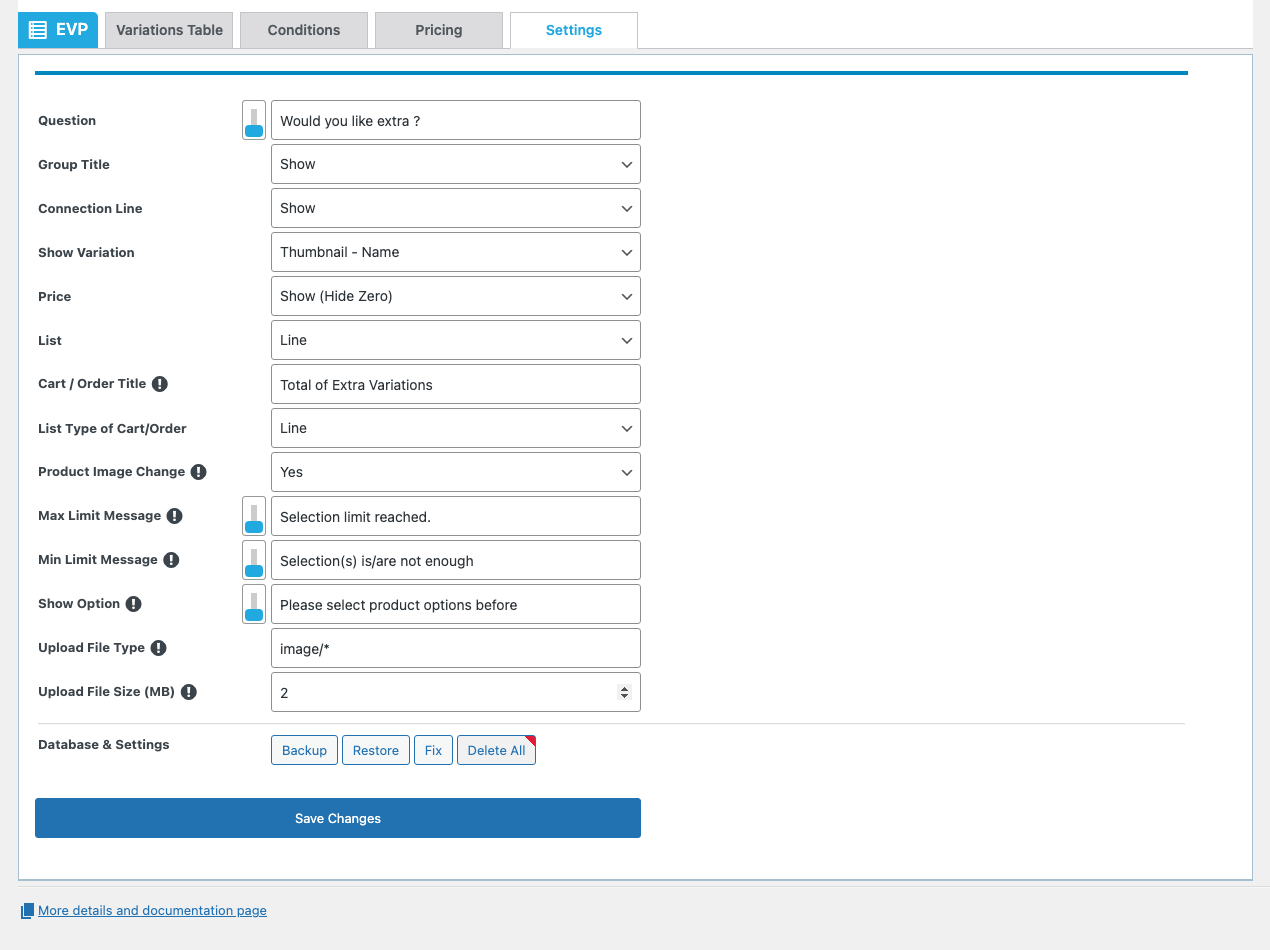**Screenshot Description: Detailed Configuration Page for EVP Variations**

The screenshot displays a detailed configuration page for EVP Variations, containing various customization settings related to conditions, pricing, and display options. The page title is prominently displayed as "EVP Variations Table Conditions Pricing Settings".

Below the title, there are multiple options presented as questions and statements, allowing the user to customize different aspects of the product variations table:
- "Would you like extra group title to show?"
- "Show connection line?"
- "Show variation thumbnail name?"
- "Price show" with an option to "Hide zero."
- "List type: list, line, cart, slash, order, title, (? mark), total of extra variations."

Further options include settings for:
- "Cart/Order line product image change" accompanied by an exclamation mark (presumably indicating the importance of the setting).
- Enabling "Max limit message," "Slider bar selection limit reach," and setting minimum limit messages, all accentuated with exclamation marks.
- Showing options with a prompt and a slider bar.
- A notification for when selections are not sufficient: "Please select product options before proceeding."

Additionally, there are options to handle file uploads:
- "Upload file type: image / * (wildcard)."
- "Upload file size limit set to 2 megabytes."

At the bottom of the page, administrative actions are listed:
- "Database and settings: backup, restore, fix, delete all, save changes."
- A link to "More details and documentation page."

The page has a clean, white background with a gray border at the bottom, contributing to a structured and user-friendly layout.

This screenshot is essential for understanding how to configure and customize the display and functionality of product variations in EVP.